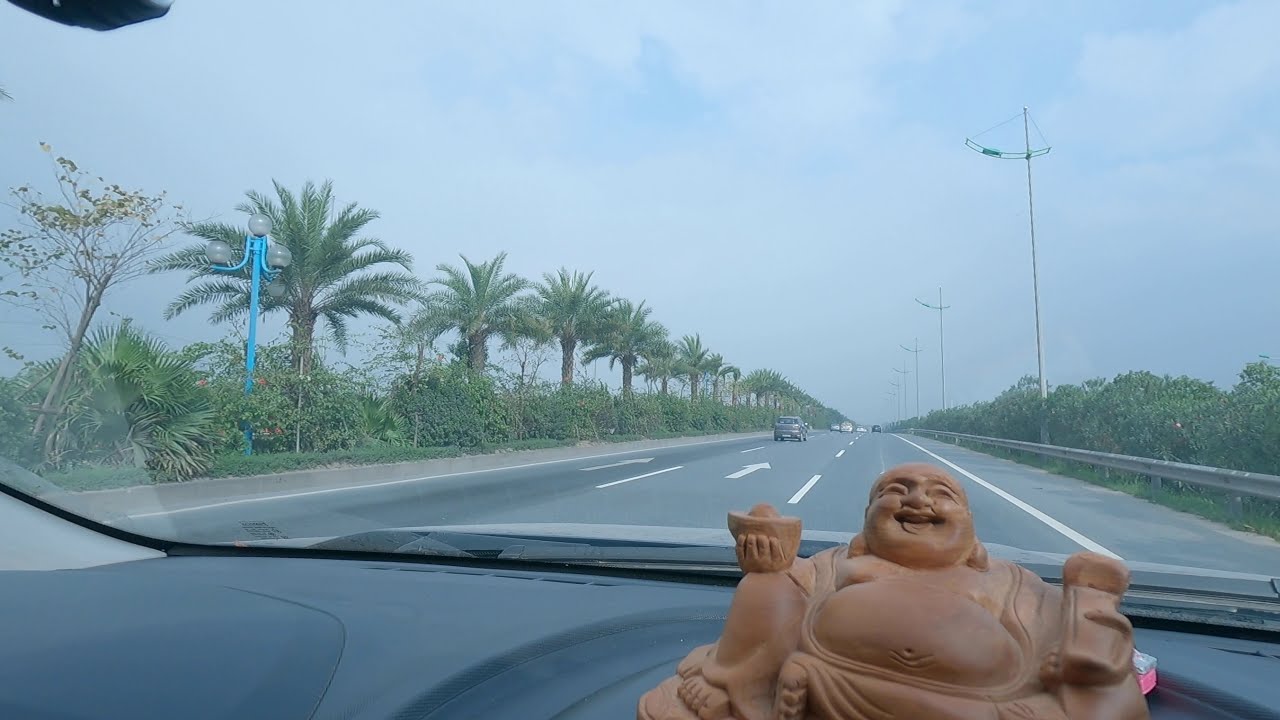The image showcases a serene highway scene from the perspective of a car's dashboard, which occupies the bottom fourth of the frame. Prominently placed on the right side of the black dashboard is a notable brown Buddha statue. Through the windshield, the road stretches ahead towards the middle of the image, spotted with a few cars and divided by white lines. Flanking the road, the right side features a metal barrier, interspersed with blue light poles and bordered by various trees and bushes. On the left side, a median filled with tropical plants, including palm trees and ferns, accompanies additional greenery and the distinct blue light pole. The top half of the image is dominated by a cloudy, bluish-white sky, emphasizing the open and inviting atmosphere of the drive. The peaceful setting of this highway, paired with the unique presence of the Buddha statue on the dashboard, captures the tranquil and reflective mood of the journey.